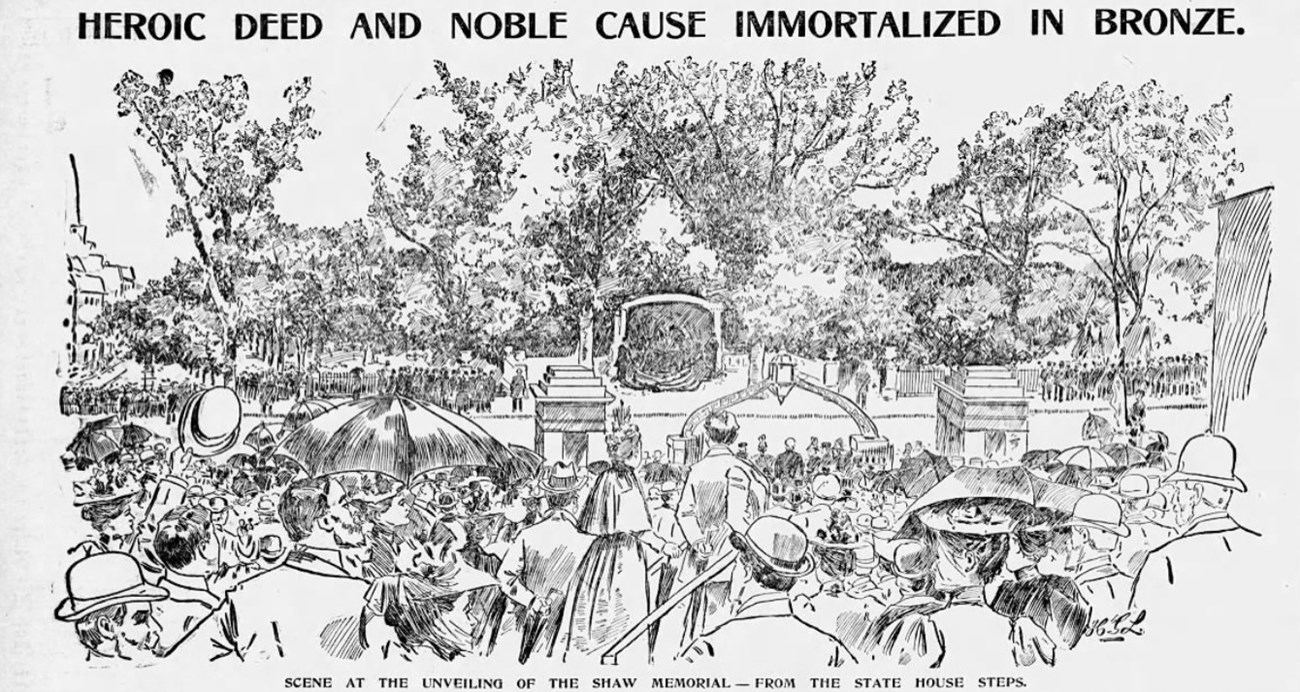This black-and-white drawing features a vintage scene, likely from the late 1800s, showcasing a crowd gathered for the unveiling of the Shaw Memorial. At the top of the image, bold text proclaims "Heroic Deed and Noble Cause Immortalized in Bronze," while at the bottom, smaller text reads "Seen at the unveiling of the Shaw Memorial from the State House steps." The attendees, dressed in period-specific attire with men in bowler hats and women in fancy hats, are depicted observing the central bronze statue dedicated to Shaw. Trees in the background partially obscure the view, adding to the serene setting of what appears to be a commemorative event held outdoors, perhaps within or near a cemetery.